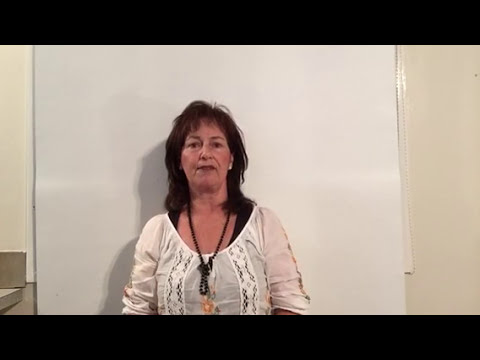This image showcases a middle-aged woman, likely in her 50s, with shoulder-length dark hair that falls softly around her face and shoulders, complemented by light wispy bangs over her forehead. Her face is oval-shaped with nicely arched eyebrows. Her expression is notably relaxed and neutral, neither smiling nor grimacing. The woman is dressed in a white knit sweater with two strips of lace down the front, layered over a black tank top, and she wears a long brown necklace in a lavalier style that drops well below the scoop neck of her sweater. The photograph, which captures her from midriff to the top of her head, places her slightly to the left of center within the frame. She stands against a blank white wall, possibly in an indoor setting like a bathroom or office space, although the setting is notably sparse, characterized only by black borders at the top and bottom of the image. The overall composition and her poised yet neutral stance suggest this could be a formal ID photo.